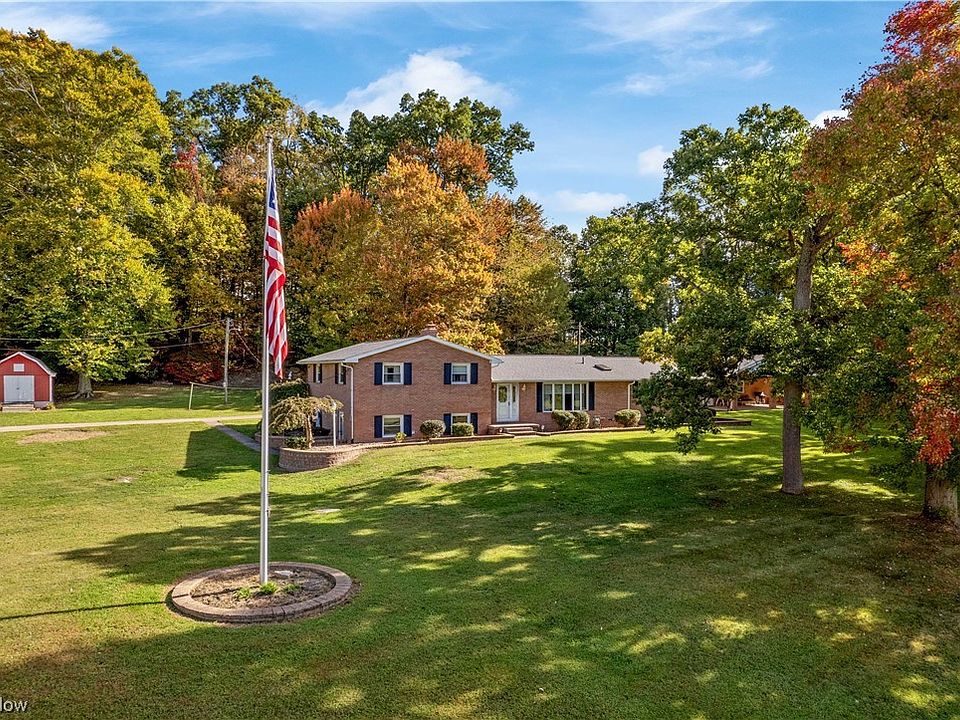The photograph captures a modest, ranch-style brick house with an orange-brown hue and light gray roof, centrally positioned in a large, well-manicured green lawn. The house features a white front door flanked by a bay window on the right and two pairs of black-shuttered windows on each floor to the left, totaling four. It is surrounded by tall trees indicating a fall setting, as the foliage showcases a mixture of green, light yellows, and oranges. Dominating the left side of the image is a tall flagpole flying a slightly turned American flag due to lack of wind. A small red shed with white doors is visible in the background to the left of the house. The sky forms a V-shape at the top of the photo, filled with wispy clouds and a puffy cloud in the center, adding to the serene atmosphere. Overall, the image highlights an idyllic, peaceful suburban scene with touches of seasonal beauty.